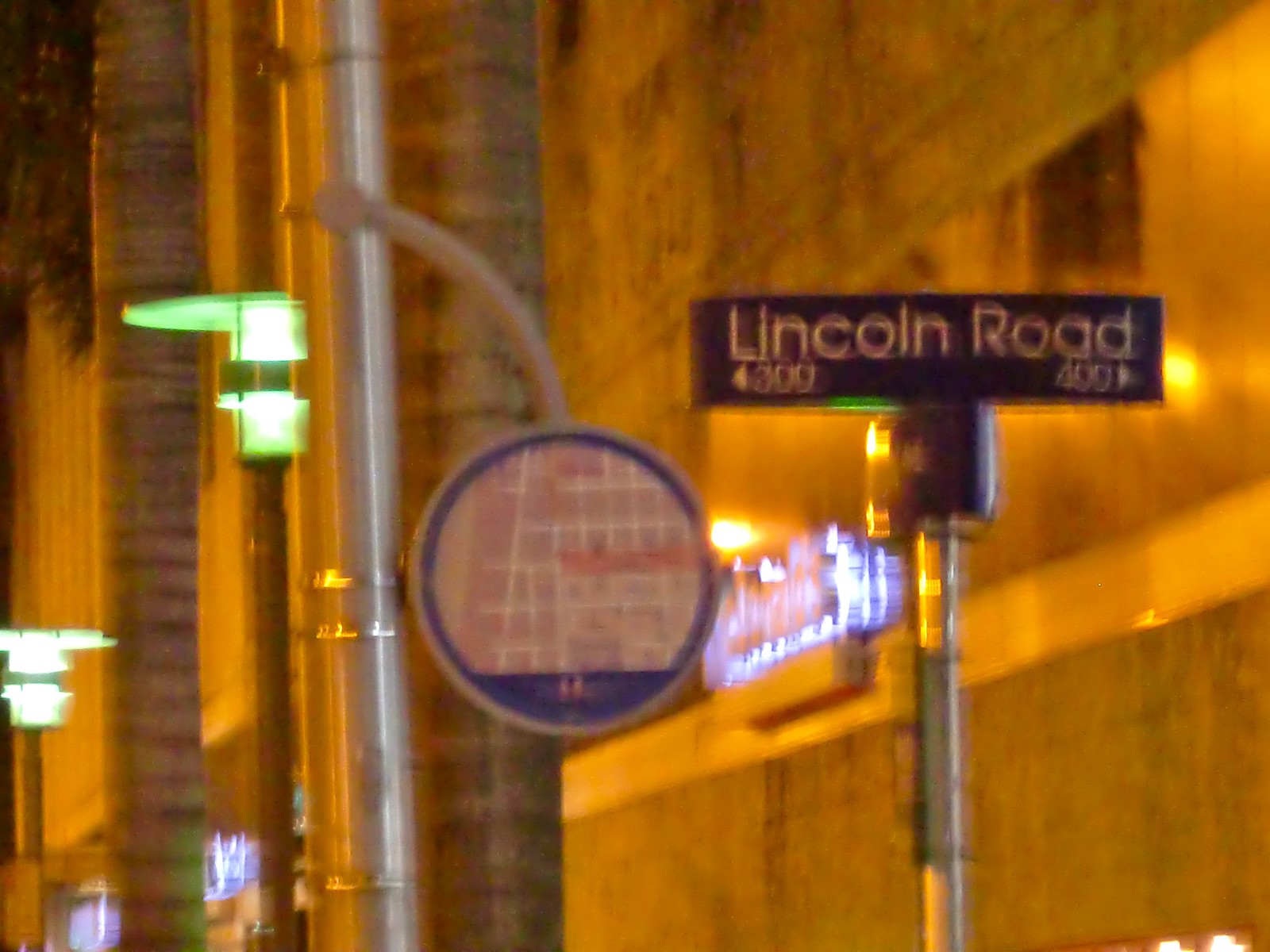This nighttime photograph, taken in an urban setting, features a close-up of a street sign on a dark blue or black cylindrical post with chrome details. The sign reads "Lincoln Road" with "300" and a left-pointing arrow on the left side and "400" with a right-pointing arrow on the right side. Attached to the pole is a circular map with a pink and dark blue outline, and a smaller blue half-circle at the bottom, which provides a bird’s-eye view of the surrounding streets. The map is held by silver rods, one bent and connecting to another. The scene includes large brick-lined pillars, some green downward-facing lights, and a white-striped wall to the right of the sign. The image also shows some green tree leaves on the left, contributing to the partly blurred and distorted nighttime ambiance. The photo has an eerie yellowish tone, complemented by various background lights including a neon sign, enhancing the urban environment.